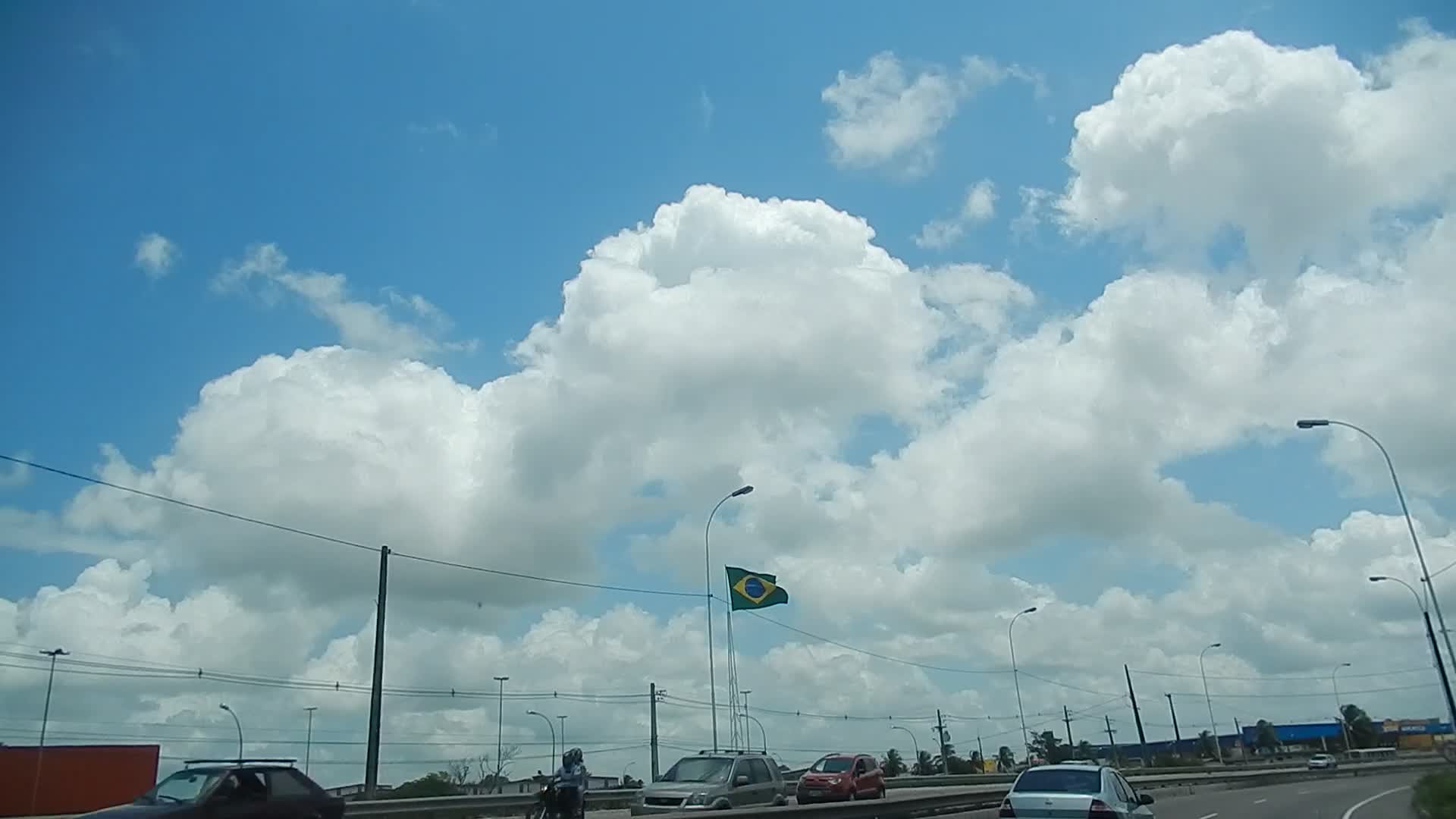The photograph captures an upward view of the sky, dominated by a cascade of beautiful, fluffy clouds set against a backdrop of brilliant blue. In the lower section of the image, a busy freeway stretches across the frame, dotted with various vehicles including a motorcycle, a red car, and two silver cars, all moving in both directions. Tall streetlights and telephone poles with electric lines trace the perimeter of the freeway, subtly framing the scene. The intended focus, however, remains on the serene and captivating sky above, contrasting with the hustle and bustle of the traffic below, offering a moment of peaceful reflection amidst the everyday rush.